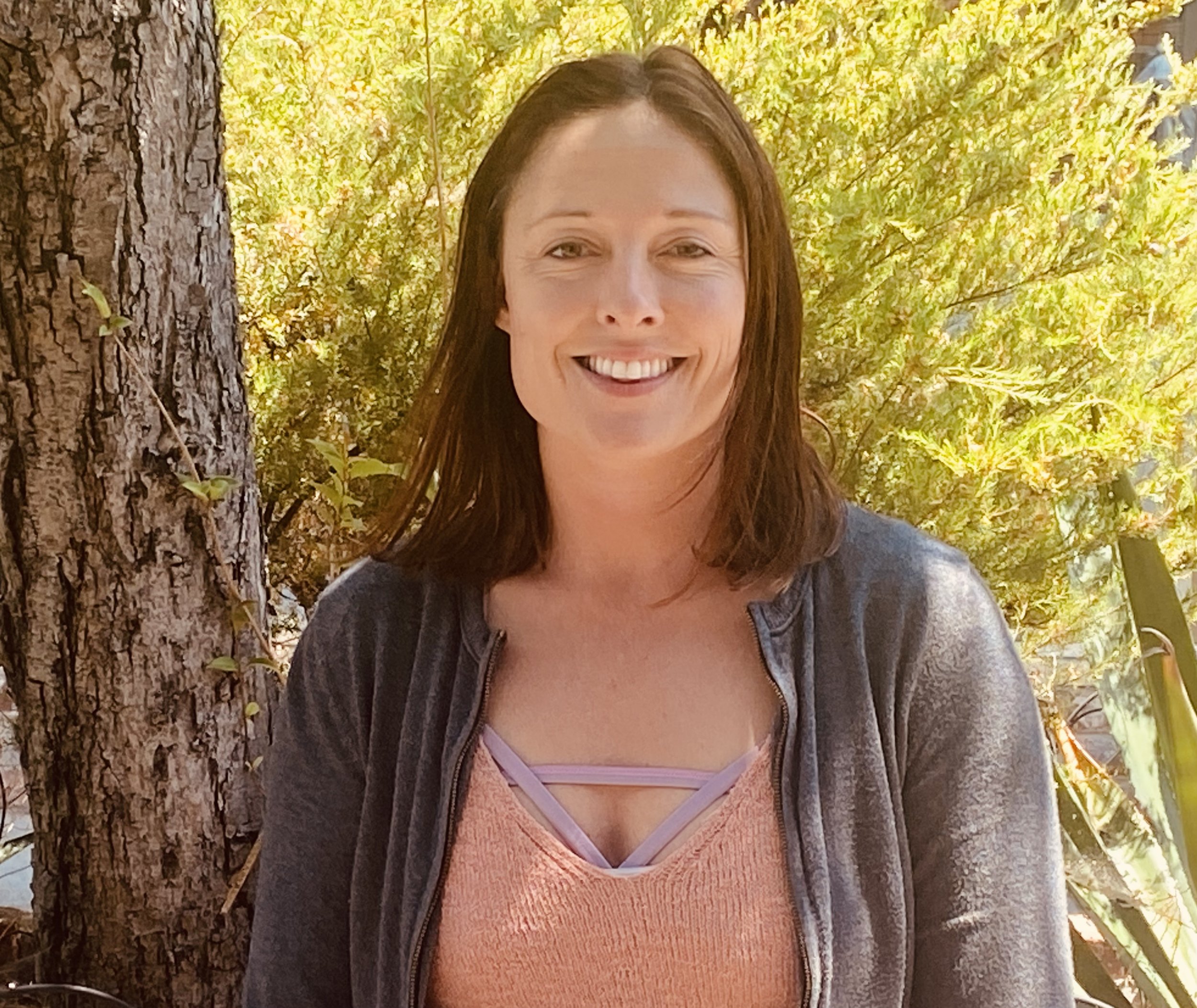In this detailed portrait taken outdoors, a woman with shoulder-length brown hair that curls at the ends is standing beside a tree trunk. She is a Caucasian female, likely in her mid-30s to early 40s, with brown eyes and a bright smile showcasing her straight, white teeth. She is dressed in a gray, unzipped sweater over a salmon-colored knit blouse, which is layered over a purple strappy garment, possibly a yoga top or sports bra. The background features a mix of greenery, with tree branches adorned with green leaves illuminated by sunlight, and additional foliage from different plants. Vines snake up the tree on either side of her, adding to the natural ambiance of the scene. She appears without makeup, highlighting her natural beauty, with thin eyebrows and some wrinkles visible around her eyes and smile lines, giving a hint of her age and adding character to her expression. Overall, the scene captures a moment of serene natural beauty with the woman as its charming focal point.